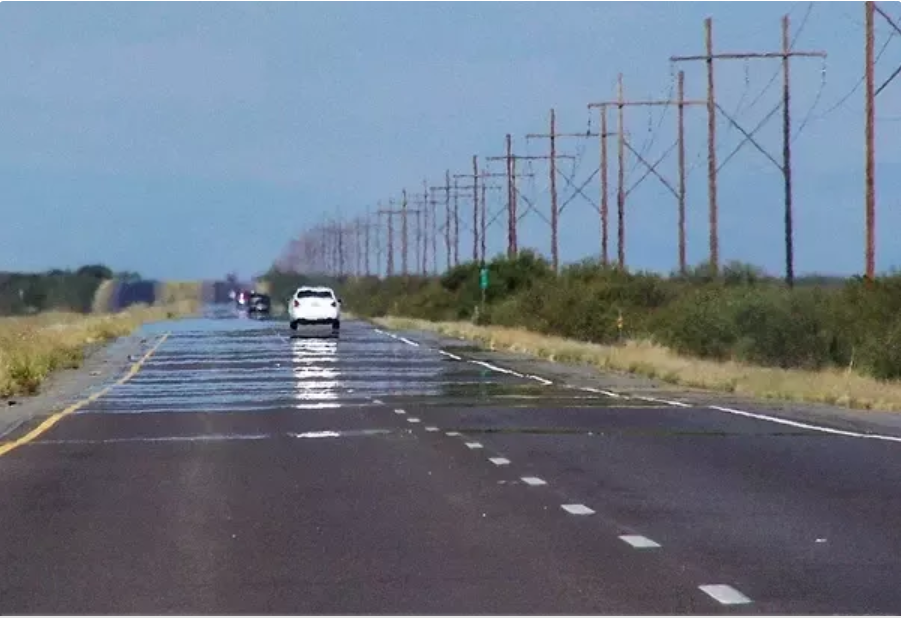This is a detailed photo of a two-lane road stretching towards the horizon under a clear blue sky. The heat shimmers off the asphalt, creating a mirage-like effect that makes the road appear reflective, almost liquid. Along the right side of the road, which is bordered by bushes and light brown grass resembling hay, there are wooden electrical poles carrying power lines that extend far into the distance. The road's center line is marked with white dashes. A yellow line is painted on the left edge of the road, while a white line traces the right edge.

Near the viewer, a white car is visible, followed by a dark-colored car further up. Ahead of them are a couple of other cars, blurry due to distance. Aside from the shrubbery to the right and some sparse grass to the left, the landscape appears relatively barren. In the far distance, a hill begins to rise, providing a subtle backdrop to this solitary stretch of highway.